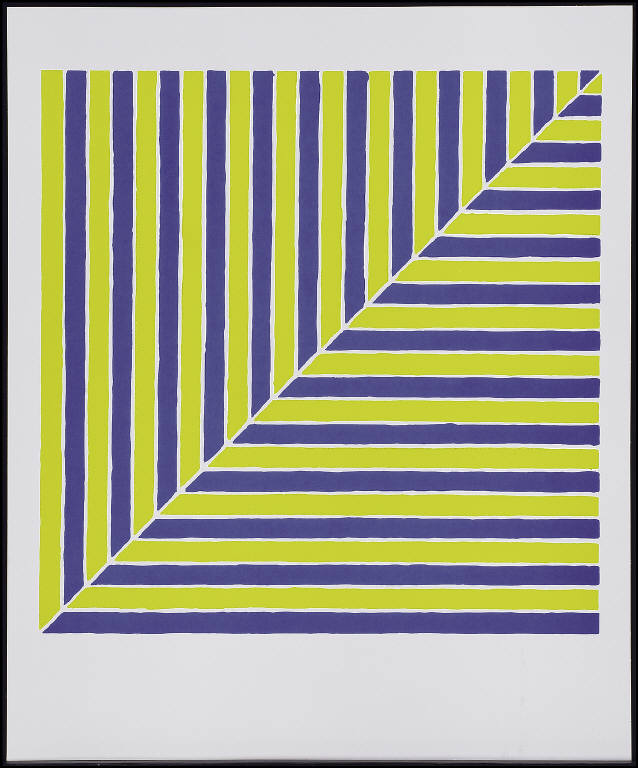This image represents a piece of abstract artwork characterized by alternating stripes of green and purple. The composition is divided by a diagonal line running from the lower left to the upper right, creating two triangular sections within a square. The upper left triangle features vertical stripes, while the lower right triangle displays horizontal stripes. These bold and evenly spaced stripes are separated by thin white lines. The entire square is set against a gray background framed by a thin black border, giving the artwork a clean and defined appearance. The design, with its distinct segmentation and vivid color contrast, forms a striking and organized visual presentation.